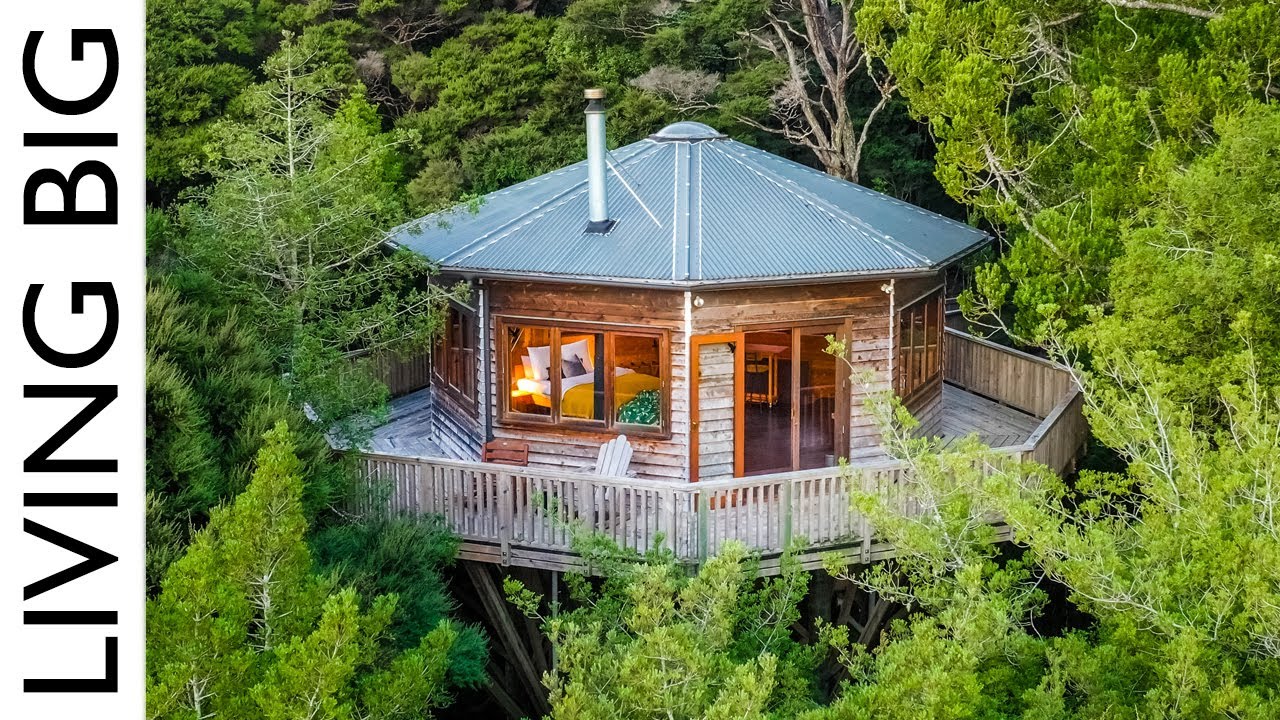The image depicts a unique octagonal wooden house situated in the midst of a dense forest, with trees, branches, and leaves enveloping and towering above the structure. The house rests on an elevated wooden platform that forms a circular deck, enclosed by a wooden railing. The roof appears to be made of green metal, featuring a cylindrical metal chimney likely for a fireplace. The siding of the house is a pale gray-brown wood, complemented by brown rectangular frames around the glass windows and glass door, which stands open. On the deck, there are Adirondack-style chairs and another wooden chair, offering a place to sit and enjoy the natural surroundings. Prominent black letters on the left-hand side of the image spell out "Living Big." The photograph is brightly lit, showcasing the clear natural setting and vibrant green foliage of the pine trees.